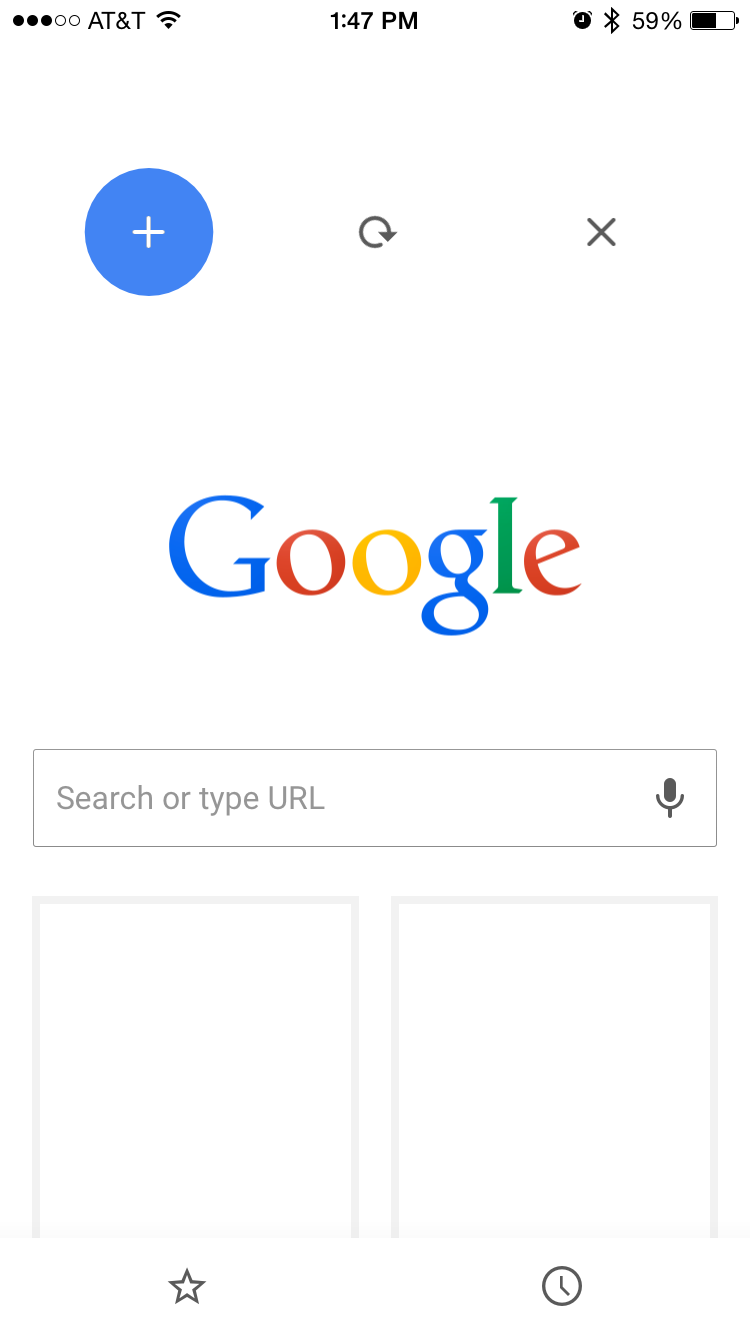This image captures a smartphone screen displaying a Google search page, indicating the device operates on the AT&T network. In the upper-left corner, there are five black dots, three of which are filled in, representing partial network strength. Adjacent to this is the Wi-Fi signal icon, followed by the time displayed as 1:47 p.m. The status bar also includes a small clock and Bluetooth icon, alongside battery information showing 59% charge with the battery icon in black.

Descending further, a white plus sign encased in a blue circle is visible, symbolizing an add feature. Centered on the screen is a refresh button, flanked by a gray X button on the right. Beneath this row is the iconic, multi-colored "Google" logo. Directly below the logo lies the search bar with the prompt "Search or type URL" and a small microphone icon situated at the far right end, enabling voice searches.

At the lower section of the image are two empty squares side by side. The one on the left features a gray star underneath, while the one on the right is marked with a gray clock icon, likely indicating bookmarks and history features respectively.